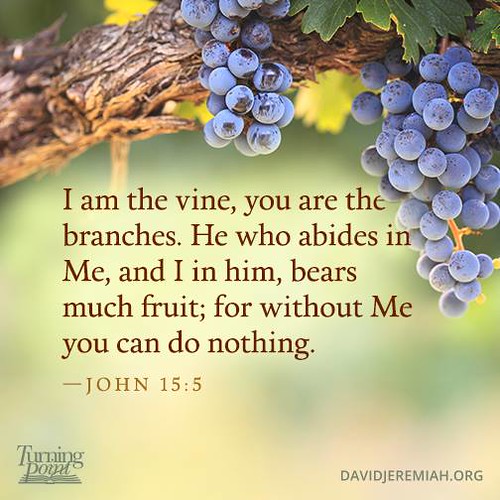This image, resembling an inspirational card or web graphic, captures a lush grapevine adorned with violet-hued grapes glistening with dew. The grapes hang from a wooden branch amidst green leaves, some tinged with yellow at their edges. The background is a softly blurred mix of green and yellow, possibly to make the overlaid text stand out. Dominating the center of the image, in a clear brown font, a Bible verse from John 15:5 reads: "I am the vine, you are the branches. He who abides in Me, and I in him, bears much fruit; for without Me you can do nothing." The verse emphasizes the spiritual message with the word "Me" capitalized. At the bottom left corner is a logo and the words "Turning Point," while the bottom right corner features the web address "davidjeremiah.org."